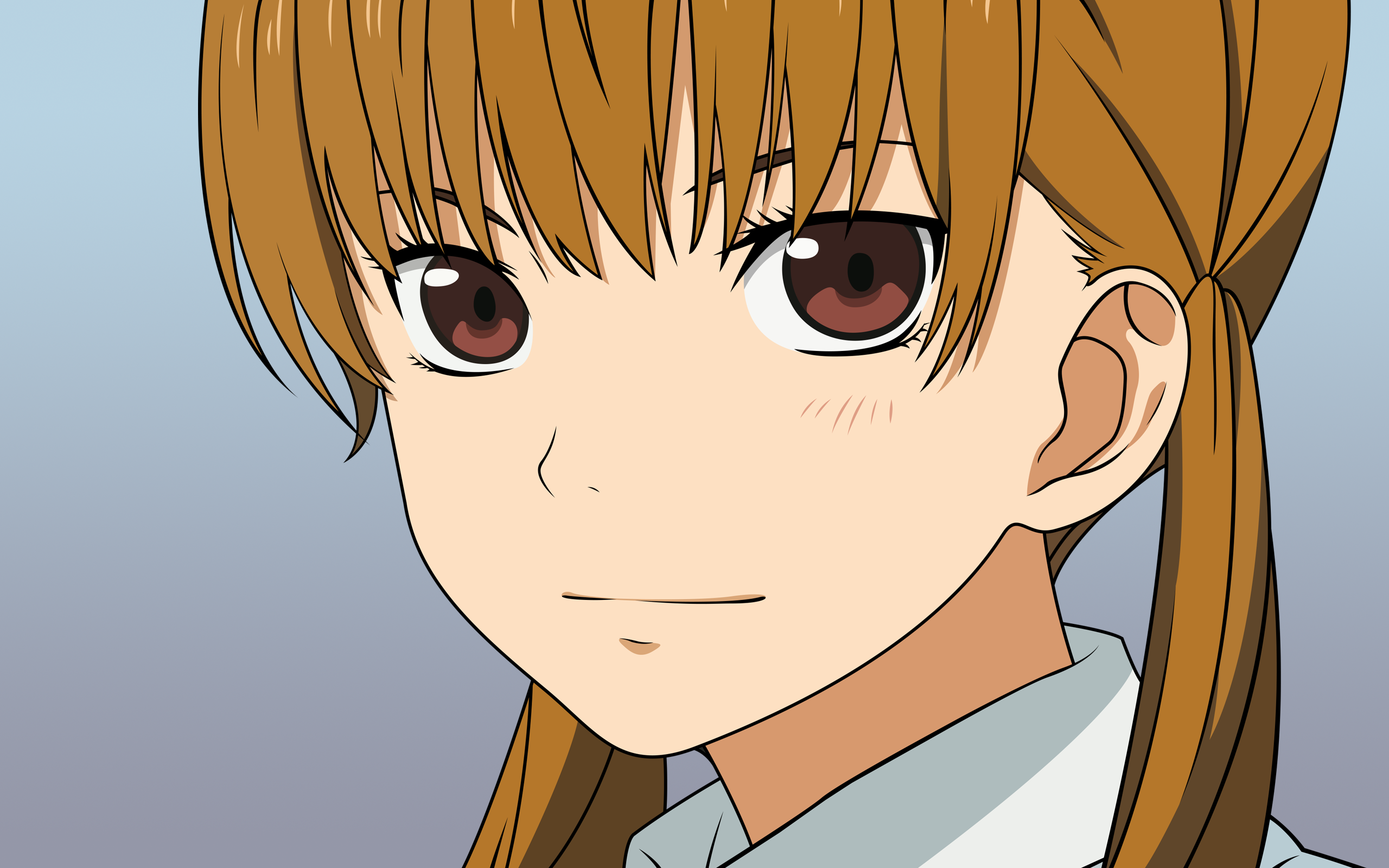The image features a young Caucasian anime girl with large brown eyes that have distinct white highlights and black pupils. Her straight light brown hair, which has a slight reddish tone, is styled in pigtails on either side of her head, with bangs that extend just below her eyebrows without covering her eyes. She is depicted wearing a collared shirt that appears gray or possibly light blue. The girl's face is turned slightly sideways to her right, but she is looking directly at the viewer. The background is blue, and the overall image is horizontally rectangular. Only her left ear is visible, and her facial features include a simple, small squiggly line for the nose and a vertical line with a small horizontal line beneath it for the mouth. Brown eyebrows and few delicate eyelashes complete her expressive anime look.